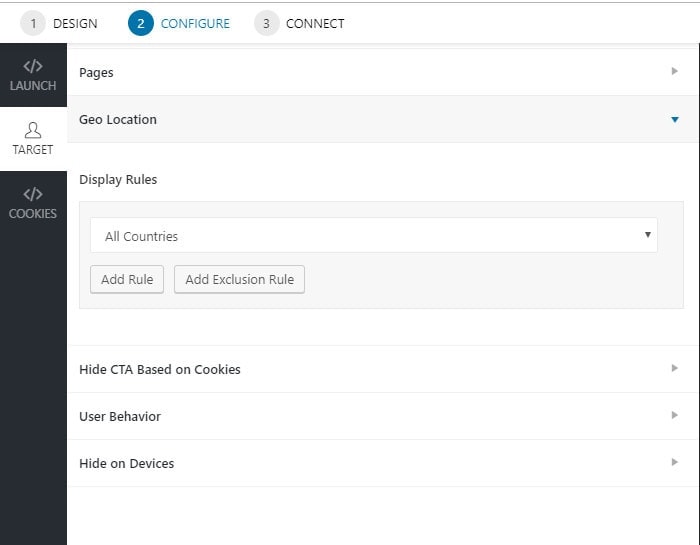This screenshot captures part of an admin or account management page, likely used by IT professionals, though key details like the company or product name are not visible. At the top of the page, set against a white background, is a series of steps displayed in gray and blue circles: 
- Step 1: "Design" (in gray)
- Step 2: "Configure" (in blue)
- Step 3: "Connect" (in gray)

On the left side is a dark gray, almost black sidebar. At the top of this sidebar, the word "Launch" is displayed in gray font next to an emblem resembling two overlapping squares pointing left and right. Below this, a white section contains the word "Target" accompanied by an icon depicting a person's head and shoulders silhouette. 

Continuing down the dark sidebar, it reads "Cookies" beside the same emblem of two triangles. To the right, a column contains various sections such as:
- "Pages"
- "Geolocation"
- "Display Rules"
- "All Countries" (alluding to dropdown options accessible via an inverted triangle on the right)

Below "All Countries," there are options to "Add Rule" and "Add Exclusion Rule" displayed side by side within a gray box. Subsequent options include:
- "Hide CTA based on Cookies"
- "User Behavior"
- "Hide on Devices"

This configuration suggests detailed customization and targeting functionalities, potentially for managing user interactions and settings.